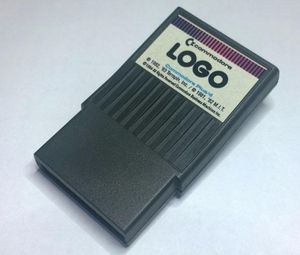The image is a digital photograph of a black cartridge laying front-side up on a light gray surface. The cartridge has a vertical rectangular shape, with the bottom part being smooth black, while the top part features textured vertical grooves. A white rectangular label is affixed to the top section of the cartridge. The label includes a prominent word "LOGO" in large, bold, all-capital letters. Above "LOGO", the label has some colored bars that are patterned purple, pink, and then purple again. Below "LOGO," there is an illegible smaller blueprint in blue and additional smaller black print, possibly detailing gears and an address. The overall color scheme of the image includes black, purple, pink, gray, and white, and there is a small shadow coming off the cartridge. The cartridge is compared to old Nintendo cartridges but is identified as longer, and despite different descriptors, looks digitally captured and is possibly a computer model or product.